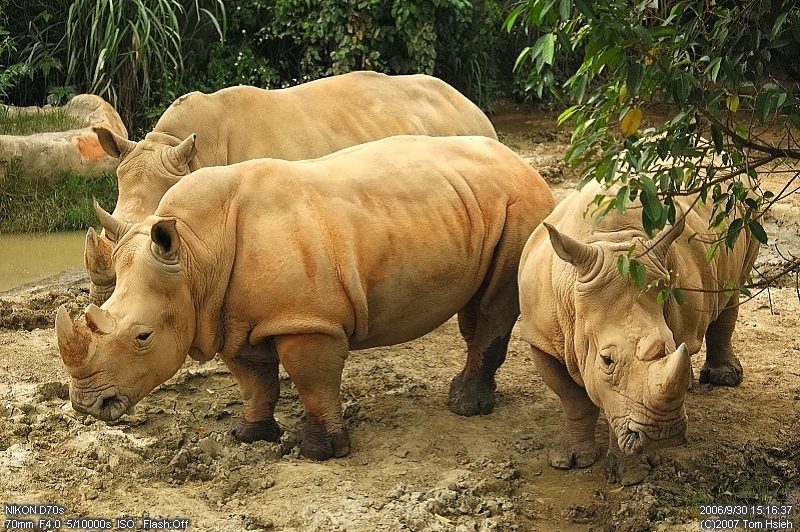This photograph captures three large white rhinoceroses within a zoo enclosure. Two of the rhinos are positioned side-by-side in such a way that the one behind is partially obscured, revealing only the top portion of its head and the tip of its nose. The third rhino is visible from the front, standing slightly behind the other two. Each rhino is characterized by its large, white horn emerging from its grey, super wrinkly nose, and their skin, which is hairless, predominantly tan, and adorned with some orange markings. Their small black eyes are encircled by wrinkled eyelids. The rhinos’ feet are caked in a dark, muddy substance, contrasting with the light tan-colored muddy surface they stand on. The background includes green shrubbery and trees with leafy branches, suggesting a lush environment. A sliver of a water source is visible on the left side. Notably, there are some grey construction elements, hinting at the enclosure setting. The image details include a Nikon d70s camera used with a 70mm focal length at f/4.0, a shutter speed of 1/5000 seconds, ISO settings, and it marks the date and time as September 30, 2006, at 3:16:37 seconds, with copyright dated 2007.